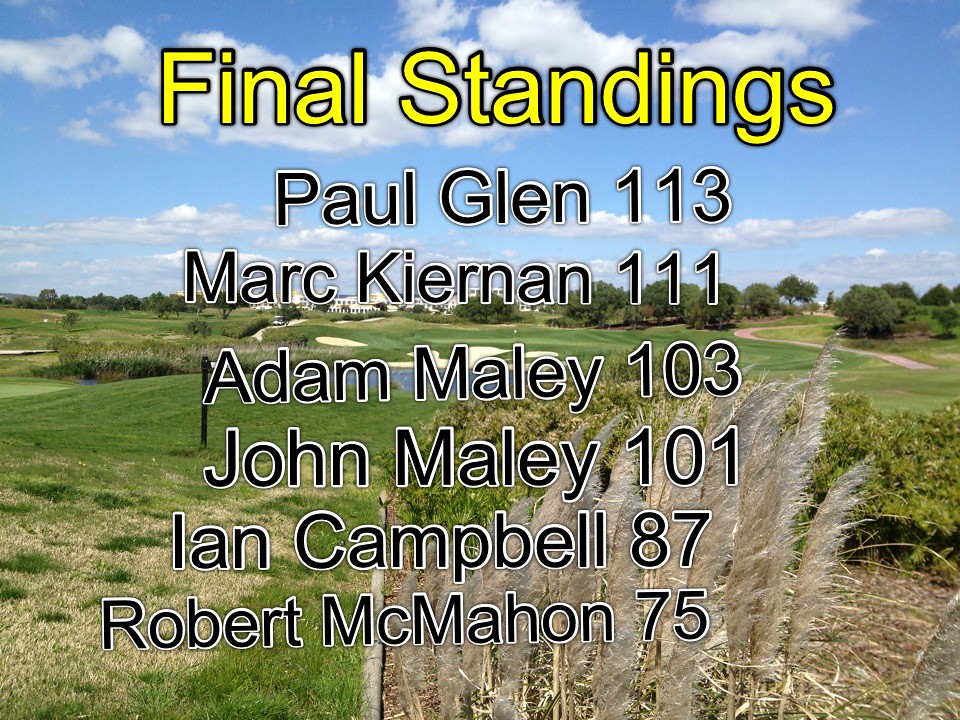The image features a scenic daytime view of a golf course under a blue sky with scattered gray and white clouds. The vibrant green grass spans much of the foreground, with patches of long grass in the corner and a hint of a marsh area accompanied by a pond. In the far distance, a few white buildings dot the horizon. Overlaying the picture, the text "Final Standings" appears prominently in yellow at the top. Below this, in black text, are the scores: Paul Glynn 111, Mark Kiernan 111, Adam Maley 103, John Maley 101, Ian Campbell 87, and Robert Mahone 75.